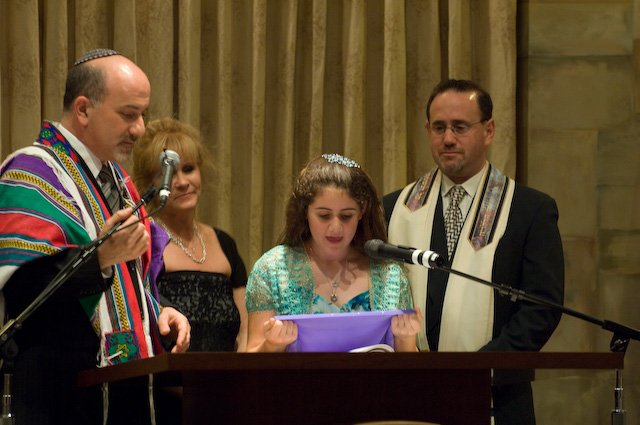The image appears to be set inside a synagogue, likely during a bat mitzvah ceremony. At the center of the composition is a young girl with brown hair, dressed in a green outfit and wearing what looks like a yarmulke. She stands at a wooden brown podium, speaking into a black microphone, while holding a purple cloth. Flanking her are two men and two women. The man on the left, possibly a rabbi, dons a yarmulke and an elaborate multicolored cloth over his black suit. Another man on the right wears a black suit with a tie, a white cloth draped around his neck, and has short brown hair. To the left of the girl is a woman with brown hair, dressed in an elegant black dress, accessorized with a necklace. Behind them is a golden-yellow curtain, set against a background with a stone wall, suggesting a religious indoor setting. The arrangement of people and objects, along with the variety of colors such as tan, gray, purple, yellow, green, red, and brown, adds to the ceremonial atmosphere of the scene.